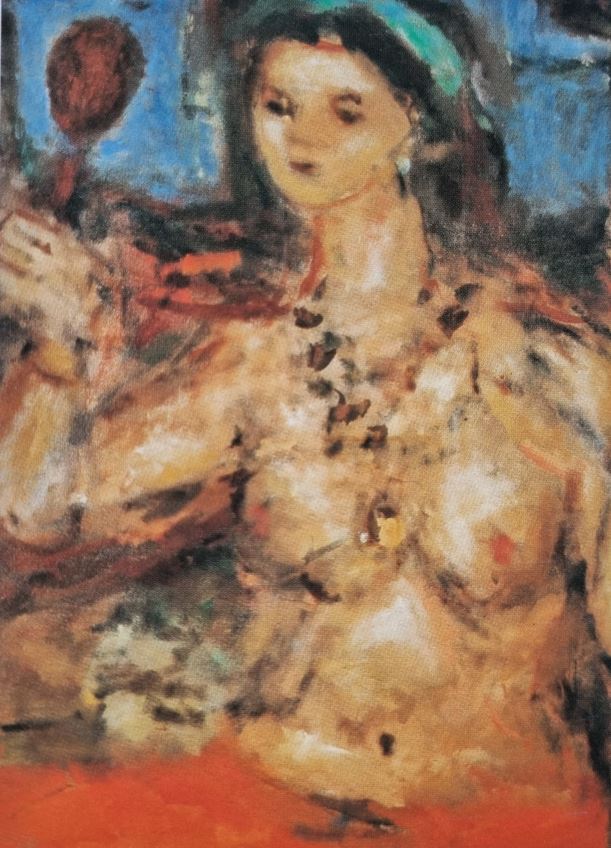This painting, executed in an impressionist style with loose and indistinct brush strokes, features a woman positioned slightly right of center. Her dark, possibly brown, shoulder-length hair is adorned with a blue or greenish ribbon that drapes from her left ear across the top of her head. The woman’s face, with distinctly wide-set eyes and pursed lips, conveys a contemplative expression as she gazes into a mirror she's holding in her right hand. Her right arm extends to the left, prominently displaying the mirror's thin handle and rounded top. She appears to be in the midst of dressing, shown naked from the waist up, highlighting her bare breasts and decorated with what seems to be a black or dark-colored necklace comprised of large brush strokes. Below her waist, she wears red bottoms that blend into the light blue background, which features bold brush strokes enhancing a dreamy, almost ethereal quality. An orange band runs horizontally across the lower section of the painting, slicing across her form just below the belly button and adding a contrasting element to the overall composition.